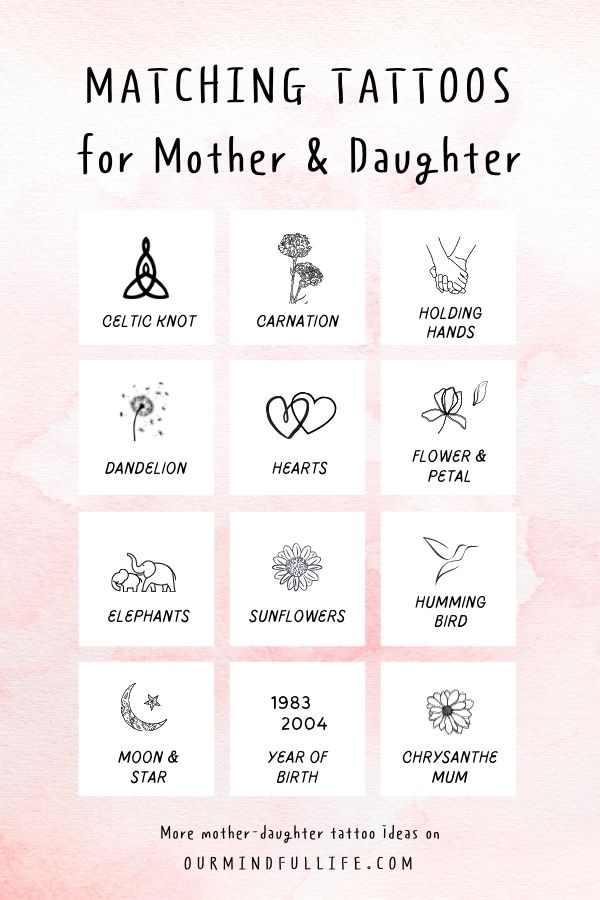Displayed on a pink and white background, this poster elegantly promotes "Matching Tattoos for Mother and Daughter" with bold black lettering. The title "Matching Tattoos" is designed in a blockish font, while "for Mother and Daughter" is written in a more scribbled style. Centrally positioned, the poster features 12 white squares, each showcasing detailed black and white illustrations of various tattoo ideas along with their titles. These tattoo designs include a Celtic Knot, Carnation, Holding Hands, Dandelion, Intertwined Hearts, Flower and Petal, Elephants, Sunflowers, Hummingbird, Moon and Stars, Year of Birth, and Chrysanthemums. Each thumbnail offers a visual preview, such as a dandelion blowing in the wind or two hearts conjoined together. At the bottom, the poster encourages viewers to discover more mother-daughter tattoo ideas at "OurMindfulLife.com".